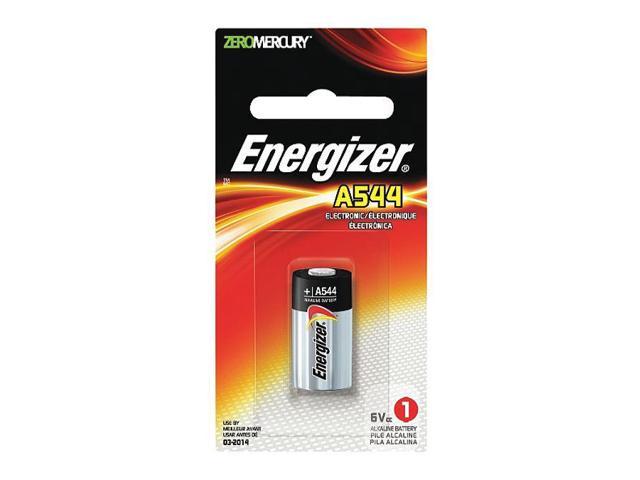The image depicts the packaging for an Energizer A544 battery, displayed against a pristine white background. The packaging design features a vibrant combination of red, black, white, yellow, and green colors. Notably, at the top left corner, the phrase "Zero Mercury" is highlighted, with "Zero" written in a green font and "Mercury" in a white font. 

The packaging also includes a small punched hole at the top center for hanging purposes. The brand name "Energizer" is prominently printed in a large, white font across the top. Directly beneath it, "A544" is distinguished in a yellow font, and the word "Electronic" is noted in white text.

In the center of the packaging is an image of the battery itself. The actual Energizer A544 battery sports a silver and black design, with the brand name "Energizer" written in black, alongside "6 volts," indicating its voltage. Additionally, the package explicitly specifies it as an alkaline battery and highlights its single pack status with a red circle displaying the number "1."